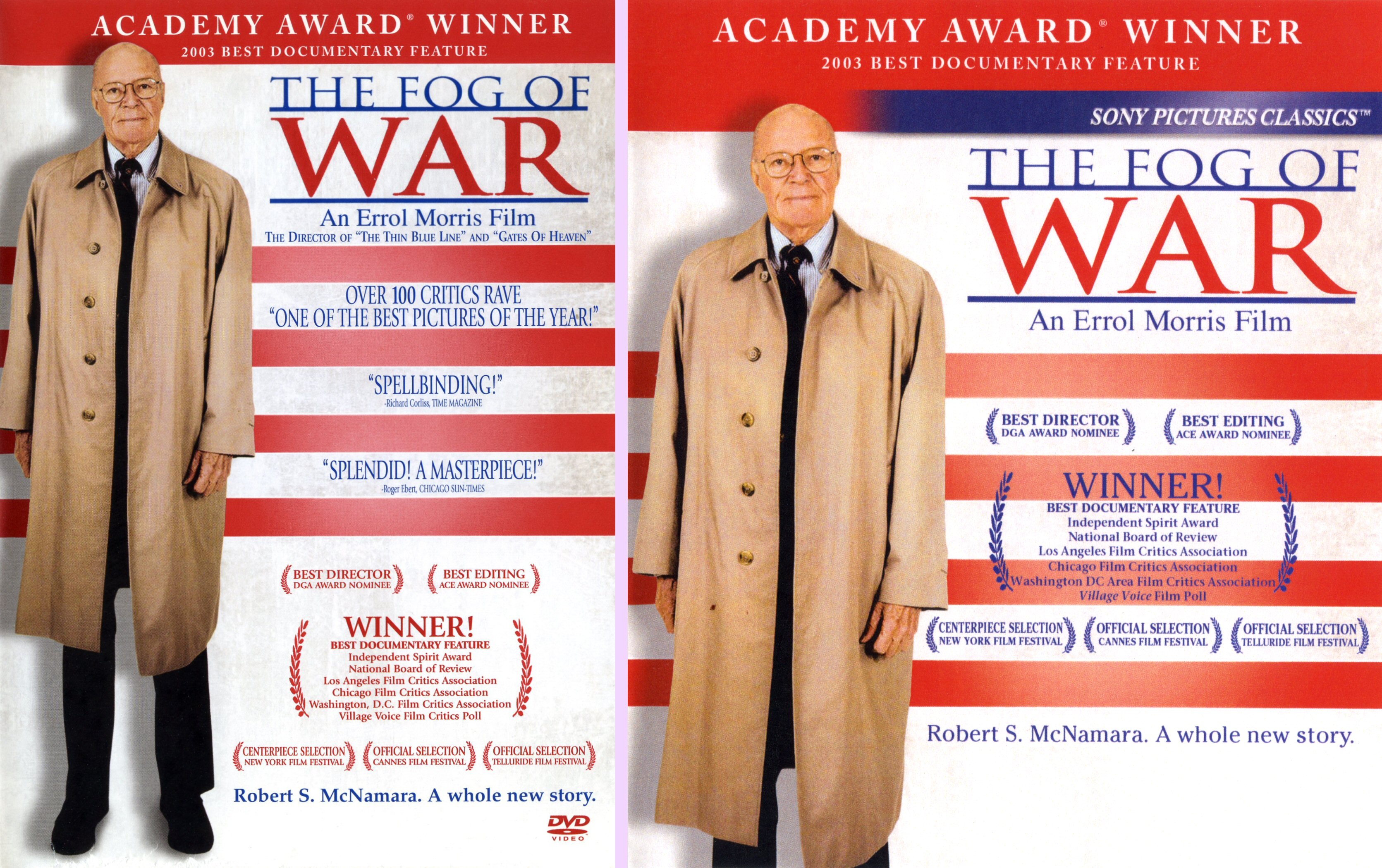This advertisement for the documentary film "The Fog of War" is designed as a split-screen image, showcasing two similar cover designs side by side with minor differences. Dominating both sides is the prominent headline: "Academy Award Winner, 2003 Best Documentary Feature." Below, the film title "The Fog of War," directed by Errol Morris, is displayed. The left side features quotes and raving reviews from over a hundred critics, highlighting phrases like "one of the best pictures of the year," "spellbinding," "splendid," and "a masterpiece." Additionally, it notes Morris's previous works, "The Thin Blue Line" and "Gates of Heaven." On the right side, accolades such as Best Director, DGA Award Nominee, and Best Editing Winner are emphasized, along with the Sony Pictures Classics logo. Both sides of the image prominently feature a distinguished, elderly bald man clad in a long tan trench coat, button-up shirt, and tie, presumably Robert S. McNamara. The color palette of the image is dominated by red, white, and blue, with hints of tan and black, creating a visually compelling and cohesive advertisement for the documentary.